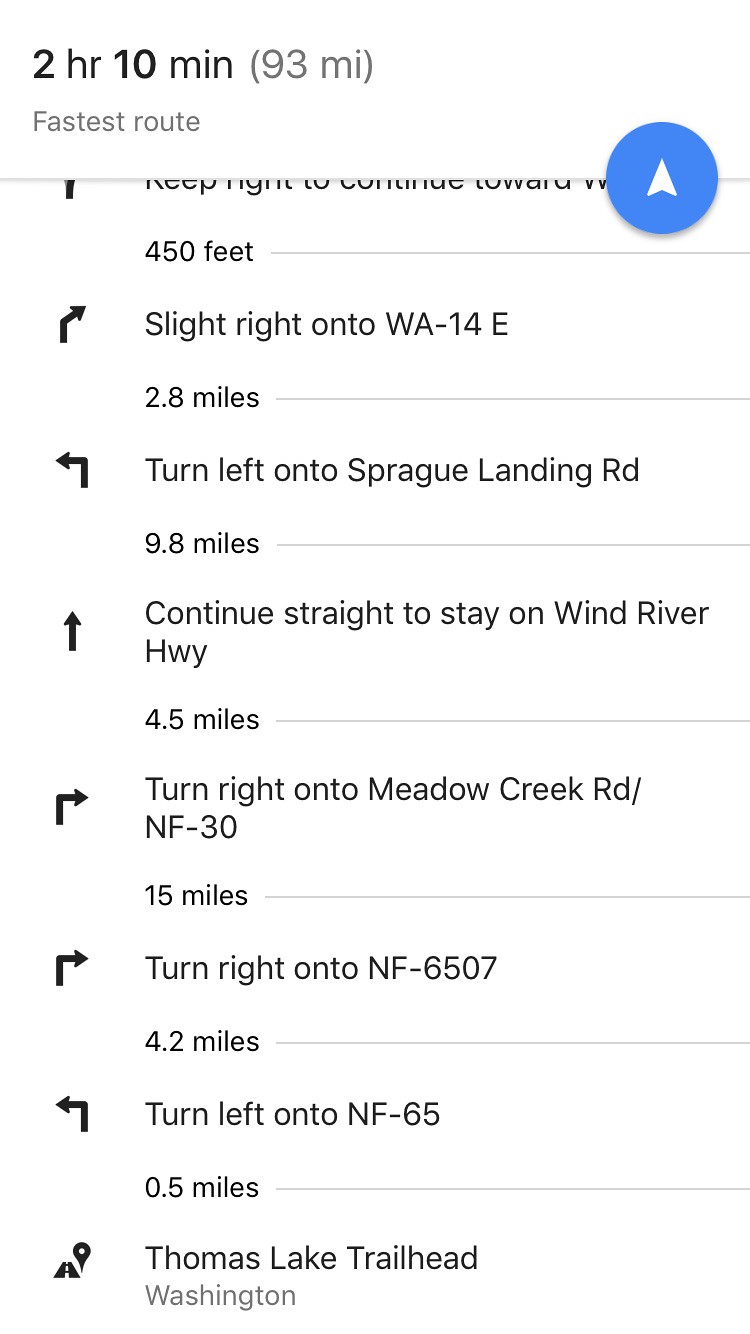This detailed image features a screenshot of driving directions, likely from Google Maps, arranged vertically. The background is white, with all text in black, except for a prominent blue circle with a white upward arrow. At the top, it indicates a travel duration of "2 hours and 10 minutes" covering a distance of "93 miles," labeled as the fastest route. The step-by-step directions include:

- "450 feet, keep right to continue toward [destination]." 
- "Slight right onto WA-14E for 2.8 miles."
- "Turn left onto Sprague Landing Road for 9.8 miles."
- "Continue straight to stay on Wind River Highway for 4.5 miles."
- "Turn right onto Meadow Creek Road (NF30) for 15 miles."
- "Turn right onto NF6507 for 4.2 miles."
- "Turn left onto NF65 for 0.5 miles."

The final destination is Thomas Lake Trailhead in Washington. Each instruction is paired with corresponding arrows, with directional arrows on the left and distances on the right, providing a thorough guide to the trailhead.